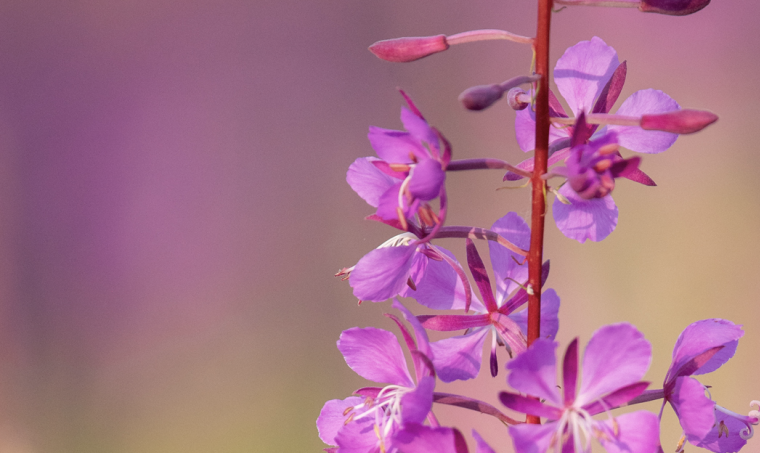This detailed color photograph, captured in a landscape orientation, features a close-up of a vibrant floral scene likely taken in a natural outdoor setting. Dominating the image is a vertical, narrow red stem adorned with several purple flowers. The flowers have distinct four-petal structures with white and light yellow stamens emerging from their centers. The blossoms are more abundant near the base of the stem and diminish toward the top, which is cut off by the frame. Notably, the upper part of the stem features a few unopened buds, with the topmost one being reddish and the one beneath it purple. The background, although blurred, illustrates a soft gradient of purple and green hues, possibly resembling a distant, out-of-focus field. This context enriches the visual narrative with more purple areas concentrated on the left side of the image, lending an artistic touch to the scene captured in photographic representational realism.